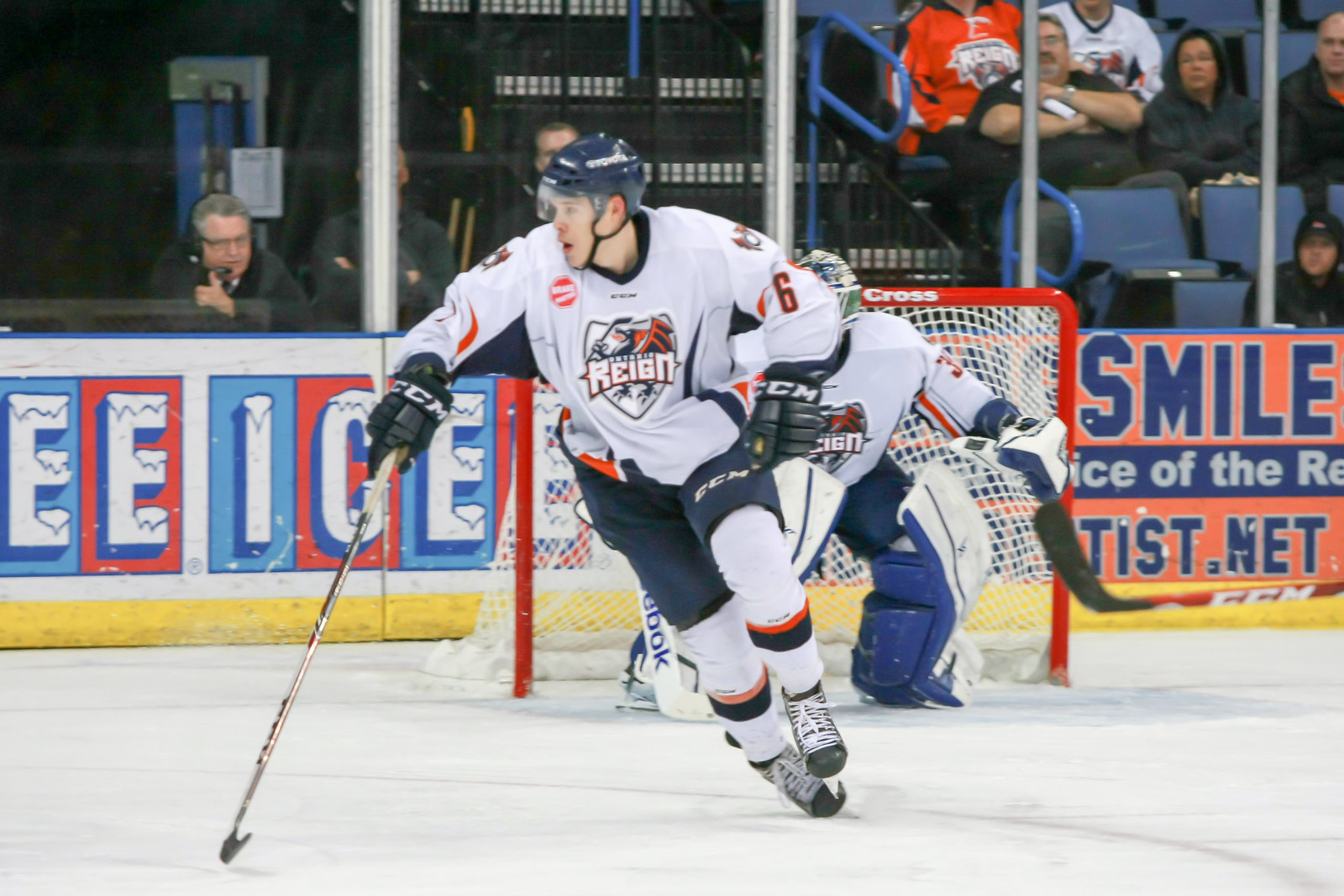In this detailed color photograph, the focal point is a professional hockey game in action. At the center of the image, a player in a white and blue uniform with black skates and gloves extends his right arm, gripping a hockey stick. His jersey is adorned with a distinctive shield logo featuring a dragon holding a hockey stick, beneath which the word "REIGN" is prominently displayed. The number six is visible on his right shoulder. He appears to be maneuvering towards an unseen puck.

Directly behind the player, the goalie, clad in matching white and blue gear, stands ready in front of the net, equipped with large white and blue pads. The net itself is a striking bright red metal frame with a white mesh. Surrounding the rink, advertisements line the white wall, including a notable blue "Icy Ice" ad and an orange sign with blue text that reads "smile."

The backdrop features a modest crowd of spectators seated behind protective glass, along with some empty blue seats and steps with blue railings. Announcers and broadcasters are stationed behind the glass on the left, adding to the bustling atmosphere of the game. The overall scene captures the intensity and vibrant details of the ongoing hockey match.